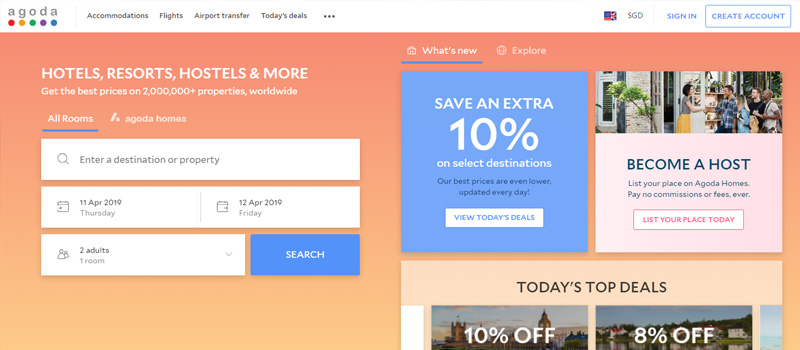The image displays a webpage from Agoda.com, a hotel booking website that provides options for booking hotels, resorts, hostels, and more. Despite not being widely recognized, the site offers a user-friendly interface for destination and date-specific searches. On the right-hand side, there is a prominent feature highlighting a discount code for an additional 10% savings. Below this section, though partially cut off, is a segment titled "Today's Top Deals," showcasing current discounts on various accommodations.